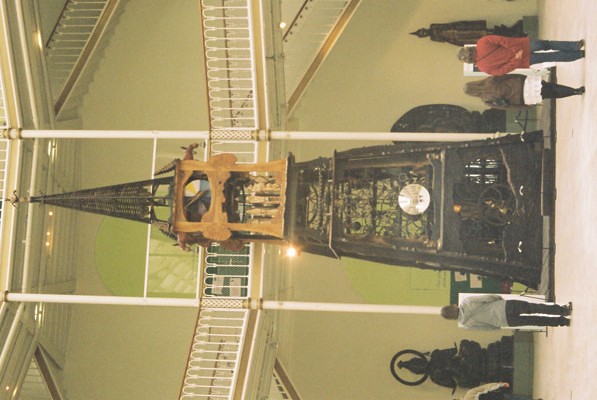The sideways color photograph captures an indoor scene within a two-story room painted in light green. Dominating the center of the image is an intricate steampunk-esque sculpture reminiscent of a mini Eiffel Tower, constructed mainly from wrought iron and rising into a triangular, pyramid shape with a large, pointy black spike at the top, capped by a golden finial. The structure features ornate white arches with brown trim and a brown central contraption, possibly an old-fashioned clock or dial, highlighted by a small, round golden plate about one-third up from the bottom. Beneath the sculpture is a mix of black and brown tones. Three individuals stand with their backs to the viewer, engaging with the sculpture—two on the right and one on the left. Surrounding this central piece are white balconies, one immediately above the sculpture and another partially visible higher up. Flanking the sculpture are figurines, adding to the room’s elaborate, somewhat Buddhist aesthetic.